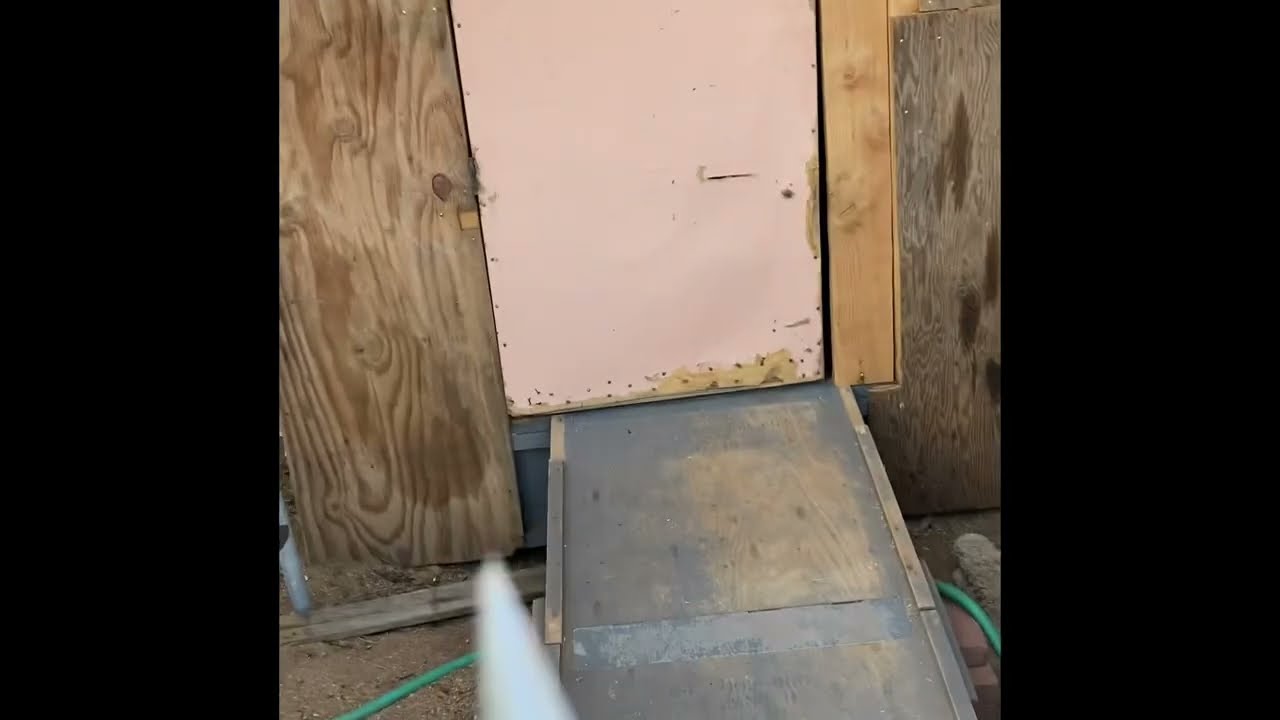The image depicts an outdoor scene with a small wooden structure resembling a shed or chicken coop. The structure is constructed from various pieces of unpainted plywood, featuring a central pinkish sliding door without visible hinges, metal handle on the right, and a key lock at the bottom. Leading up to this door is a plywood ramp, supported by red bricks and an additional two-by-four at the base. Beneath the ramp, a green garden hose runs across a muddy, rock-strewn ground. The overall environment suggests neglect and disrepair, with a visible gap beneath the wall hinting at further deterioration.